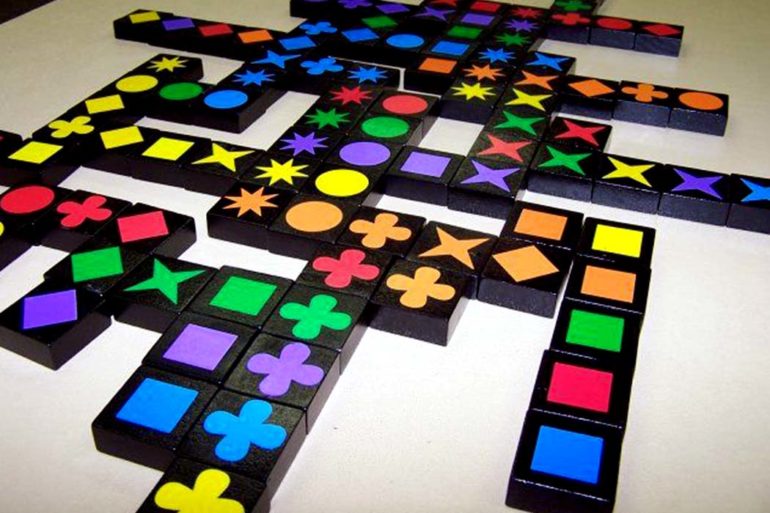The image depicts a collection of black square tiles laid out diagonally across a cream or tannish surface. These tiles cover nearly the entire image area and are arranged flat, reminiscent of a game such as dominoes. Each tile features a distinct shape, including squares, diamonds, four-pointed stars, four-leaf clover-like shapes, triangles, and circles. The shapes are displayed in a variety of vibrant colors: yellow, blue, purple, green, red, and orange. The scene suggests a playful, organized layout that could be found in a child's room, with the colorful, patterned arrangement of tiles creating a visually engaging and structured composition. There is no text present anywhere in the image.